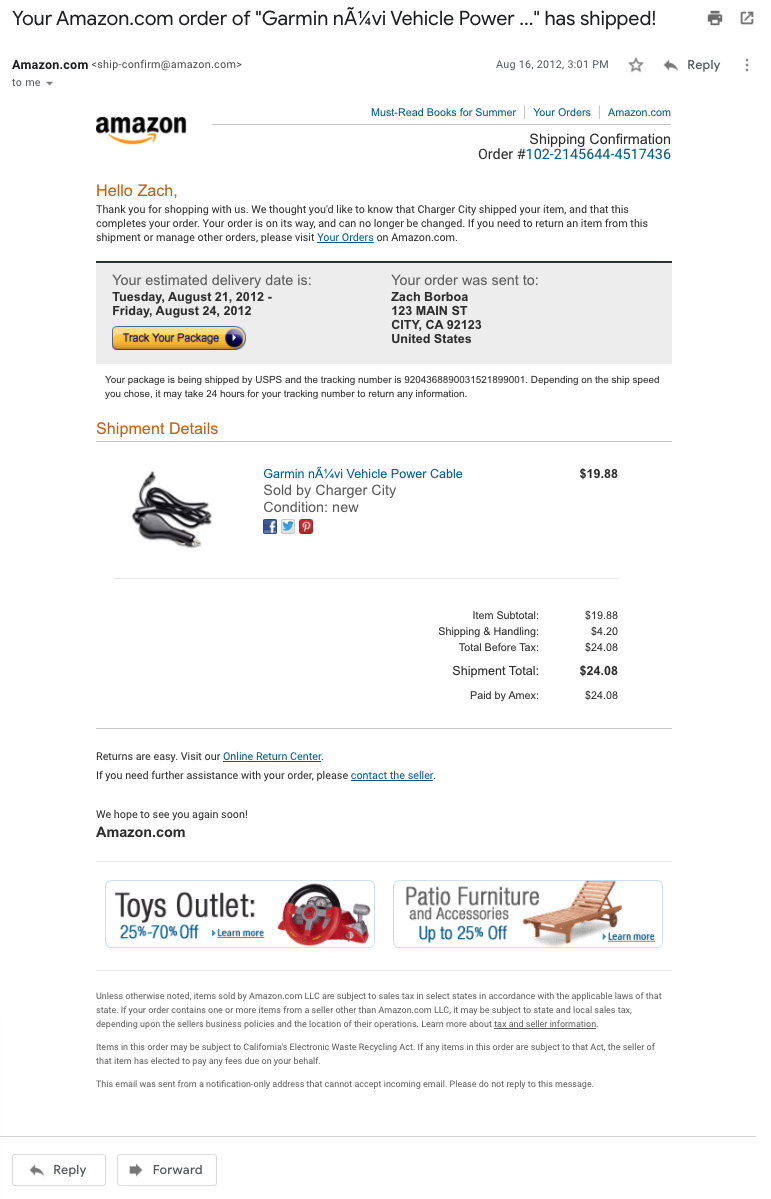This detailed caption describes an email notification from Amazon confirming the shipment of an order and provides specific details from the email's content and layout:

---

The image depicts an email confirmation from Amazon, titled "Your Amazon.com order of 'Garmin NA 1/4th Bi Vehicle Power...' has shipped." At the top, there's a black navigation bar with "Your Amazon.com order of 'Garmin NA 1/4th Bi Vehicle Power...' has shipped" displayed prominently. Below this, the sender is shown as "amazon.com," with the email address "ship-confirm@amazon.com" and a timestamp of "August 16, 2012, 3:01 PM."

On the left side beneath the header, the Amazon logo is visible, and to the right, a banner reads "Must Read Books for Summer." The main body of the email greets the recipient with "Hello Zach," followed by a thank you message: "Thank you for shopping with us. We thought you'd like to know that Charger City shipped your item and that this completes your order. Your order is on its way and can no longer be changed. If you need to return an item from this shipment or manage other orders, please visit Your Orders on amazon.com." The phrase "Your Orders" is hyperlinked in blue.

The email provides an estimated delivery date range of "Tuesday, August 21, 2012, through Friday, August 24, 2012." A yellow button with blue font labeled "Track your package" is included below this information. Lastly, the order shipping address is listed as:

Zach Borbo  
123 Main Street  
City, California 92123  
United States

This clear structure and detailed layout ensure the recipient has all the necessary information regarding their shipment.

---